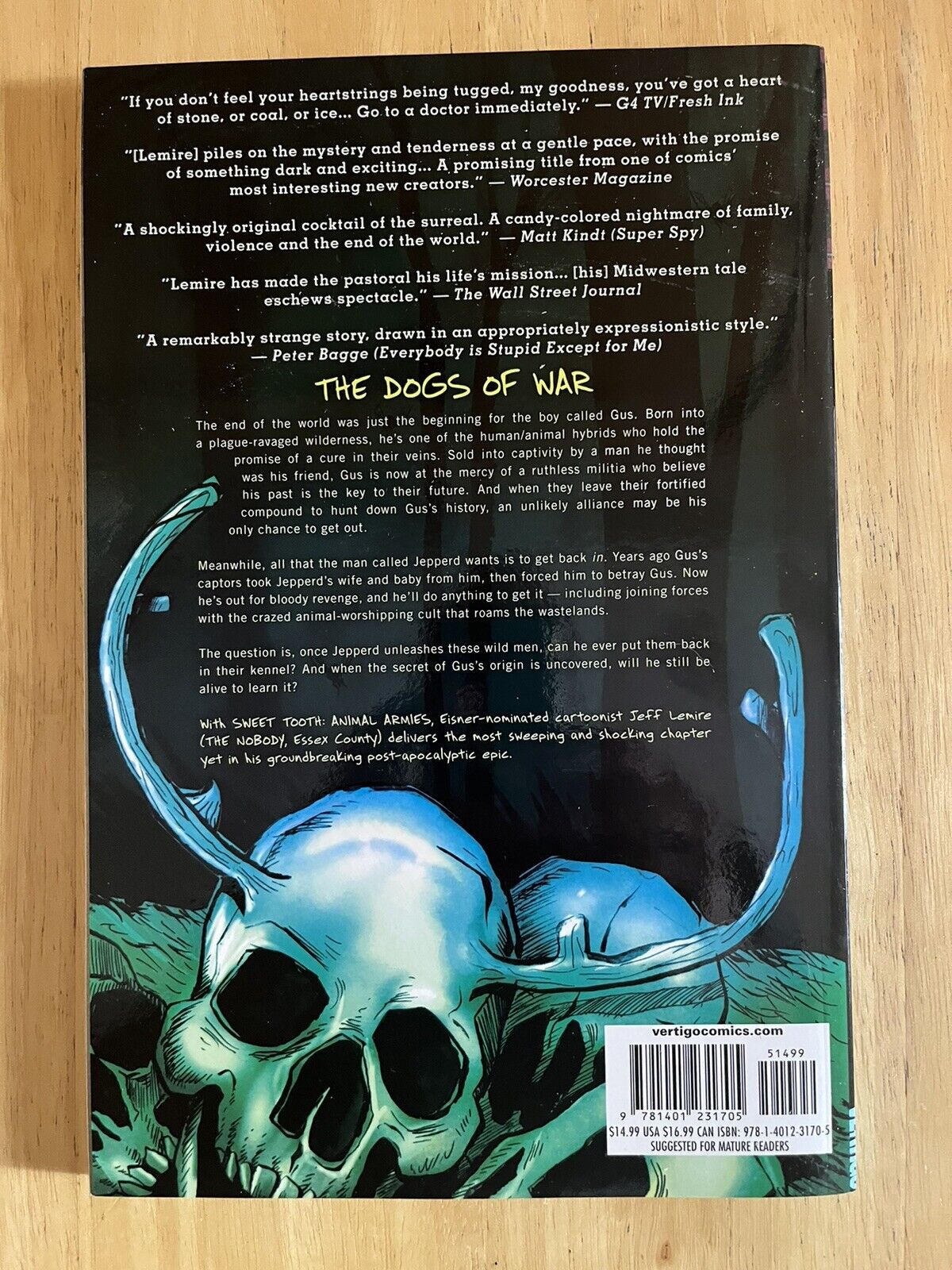The back jacket of the comic book *Sweet Tooth* features a striking design set against a wooden surface. The majority of the background is black, transitioning to green and blue hues towards the bottom. Prominently displayed at the bottom center are two skulls with antlers; one skull is predominantly blue with green around the eyes and mouth, while another peeks out from behind it on the right. A white UPC label is situated in the bottom right corner, and at the very top is the website vertigocomics.com.

The upper portion of the back cover is filled with various reviews and blurbs in white text, praising the work. Notable publications such as the Wall Street Journal and Worcester Magazine contribute to the commendations. Encircled in yellow text, the title "The Dogs of War" stands out in the middle above the descriptive text about the comic's storyline. This particular edition describes a post-apocalyptic tale involving a boy named Gus, who is a human-animal hybrid sought by a ruthless militia. It also introduces Jepperd, a man driven by revenge, who enters an uneasy alliance with a savage cult. The storyline promises tension and excitement, building on Jeff Lemire's reputation as a remarkable storyteller in the graphic novel world.